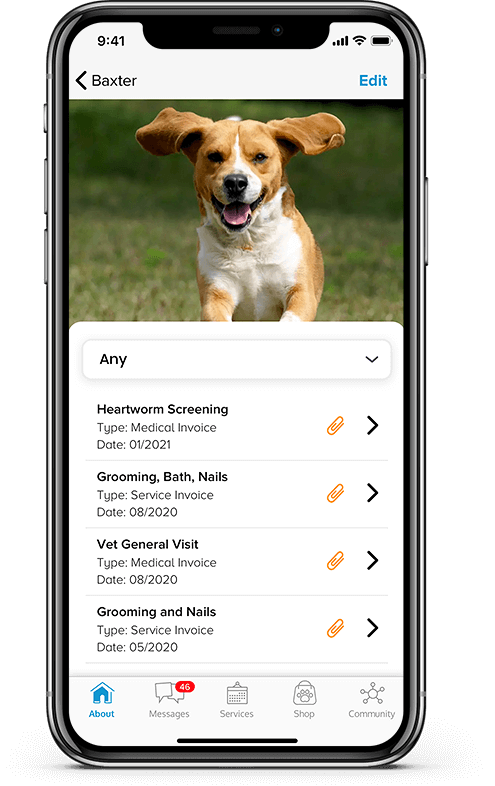The image displays an iPhone screen showcasing a pet-related application, likely focused on dog adoption or dog walking services. The app has a clean, white background. Prominently featured at the top of the screen is an image of a running dog against a backdrop of vivid green grass. The dog's name, "Baxter," is displayed on the top left corner of the screen, with an "Edit" option on the top right.

Below the header, there is a drop-down menu labeled "Any." Further down, there are four additional menu items: "Heartworm Screening," "Type: Medical Invoice" with a date and an attachment icon next to it, "Grooming: Bath, Nails" with another attachment icon, "Vet General Visit," and a repeat of "Grooming: Nails."

At the bottom of the screen, five navigation options are provided. The highlighted "About" option is in blue, as this page is currently open. Next to it, the "Messages" option shows a red notification badge indicating 46 unread messages. Following this are the "Services," "Shop," and "Community" tabs.

The layout is user-friendly, focusing on Baxter's profile and various pet care services.